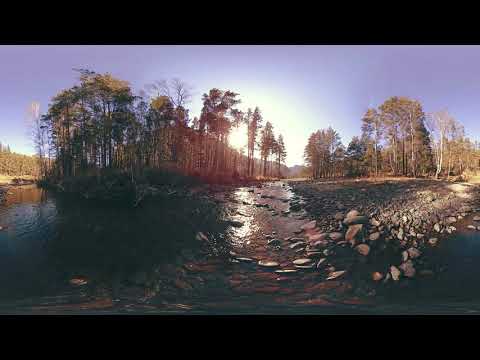The photograph depicts a tranquil outdoor scene that could easily be from a nature park or a national forest. The bottom half of the image is dominated by a rocky shore composed of brown and tan rocks, with some water creeping up onto them. The water appears dark, almost black or purplish in certain areas, indicating a low tide or just a low water level in general. Some of these rocks are also visible in the water. 

In the upper part of the image, a lush green tree line stretches from left to right, featuring tall, slender trees, some of which have a reddish hue from the sunlight. Behind this verdant backdrop, the sky is a clear blue with no clouds in sight. At the center of the photograph, nestled behind the trees, the sun is either rising or setting, casting a soft light that enhances the scene's natural beauty. There are black bars at both the top and bottom of the photograph, running horizontally from one side to the other, possibly indicating a panoramic shot.